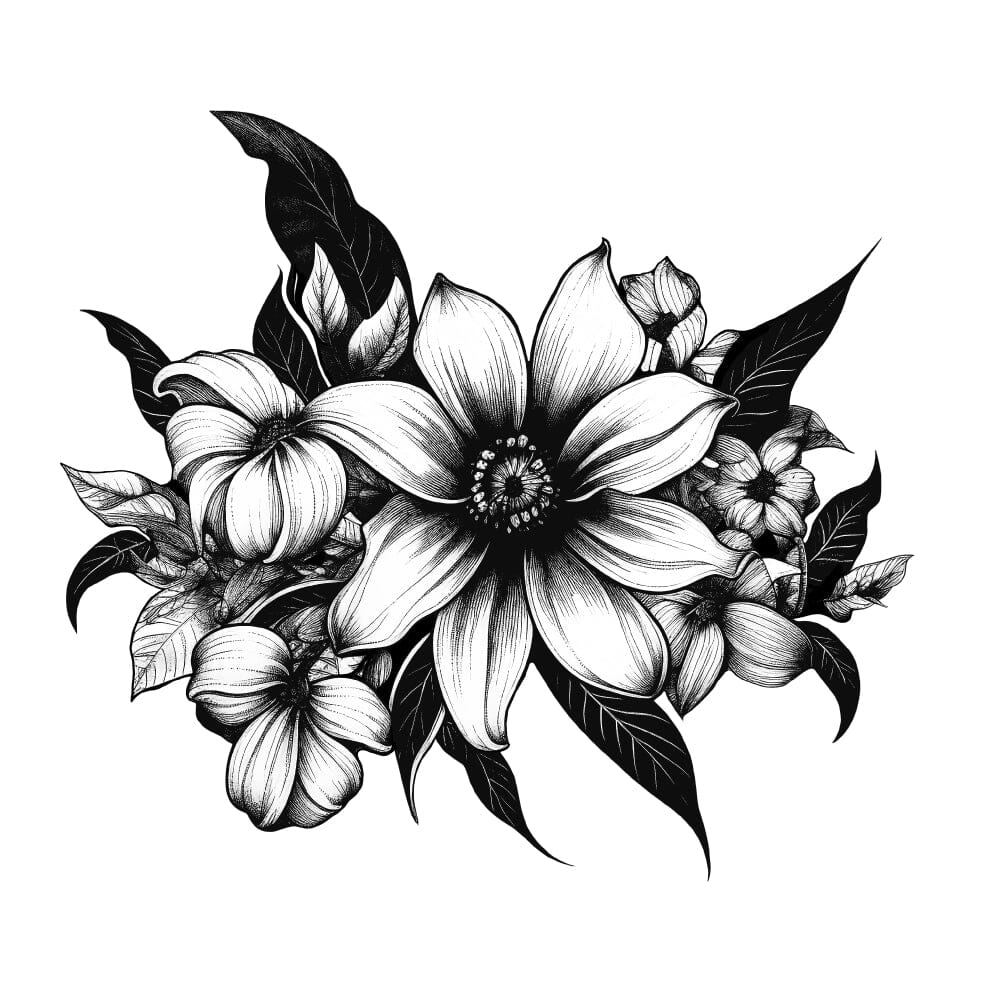This intricate black and white illustration features a series of delicately drawn flowers and leaves set against a pure white background. The composition is framed by an array of slender, dark black leaves that form an almost oval shape, tapering to elongated points at either end. Each leaf is detailed with fine white line work that intricately captures the veining, adding a sense of depth and texture. At the center of this leafy border, several white flowers take focus. Each flower has a dark center filled with small, white seed-like details, surrounded by white petals that radiate outward in a sunflower-like fashion. Black line work traverses these petals, enhancing the texture and natural flow of the flowers, creating a harmonious balance between the elements on the white canvas.